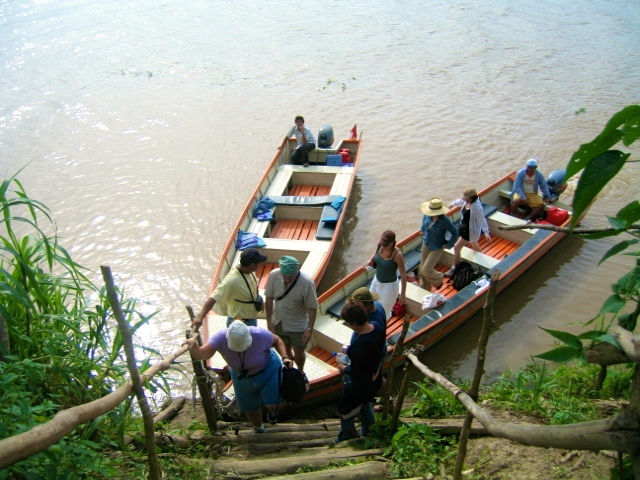The photorealistic image depicts a group of tourists, predominantly white and casually dressed, arriving at a remote riverbank on two long boats. Each boat is equipped with five seats, cushions, and an outboard motor, with one person guiding each boat. The scene takes place in what appears to be Southeast Asia, judging by the lush, dense foliage and the dark brown color of the water, indicative of a river. The boats have docked by simply touching their noses to the muddy, grassy bank. The tourists are shown climbing up a steep inclined path that serves as a makeshift dock. The path is constructed from logs embedded in the dirt, forming crude steps, with handrails made of curved, twisted branches running alongside. A woman in a purple shirt and black shorts is visible in the foreground, ascending the stairs. The overall setup includes simple, rustic elements designed to enhance the remote, adventurous atmosphere of the location.